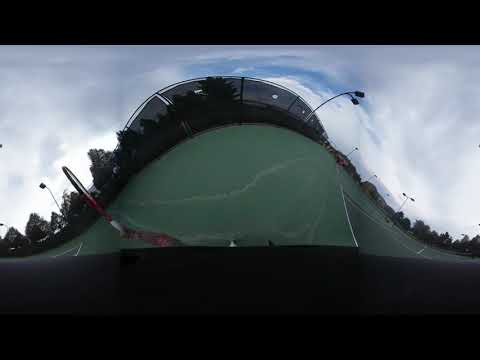The image depicts a scene captured with a wide-angle or fisheye lens, resulting in a slightly distorted, curved perspective. The setting is a tennis court with a smooth, bright green surface that looks tiled. Surrounding the entire court is a tall black fence that curves due to the lens effect. Dark green trees line the outside of the fence, which might be softly rustling in what appears to be an impending rain. Overhead, the sky is cloudy and gray, suggesting that rain could soon fall. 

On the left side of the image, an individual holds a tennis racket. The racket features a white grip, a red base, and a black top. The net of the tennis court is also visible on the right edge of the image, supported by yellow posts. Scattered lampposts around the court, each topped with two lights, add to the scene. Despite the overall blurriness and low quality of the image, these details provide a clear sense of the environment captured.